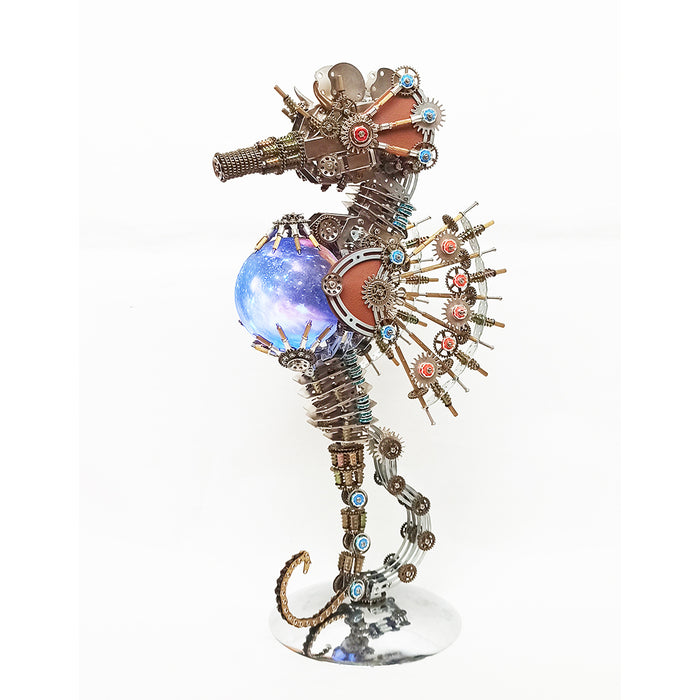The image depicts a digitally created seahorse with a distinctive steampunk aesthetic. The seahorse is meticulously crafted from various metal pieces, evoking the look of an intricate mechanical sculpture. Its tail curls upwards at the front, featuring a silver metal bracing adorned with brass cogs and gears, reminiscent of components from electronic devices. The most striking feature in the midsection is a large, circular gem-like structure, shimmering in hues of purple and blue with white speckles, resembling a miniature galaxy. The back of the seahorse is lined with a spine composed of gold parts with bronze cogs, interspersed with red center gears. The head is designed to appear metallic, with a bronze-colored tube as the nose and an array of silver and bronze pistons coupled with gears. Its eyes are made of gears with blue and red centers, enhancing the detailed and complex appearance. The overall palette of the seahorse combines brown-bronze tones, enhancing its steampunk vibe.